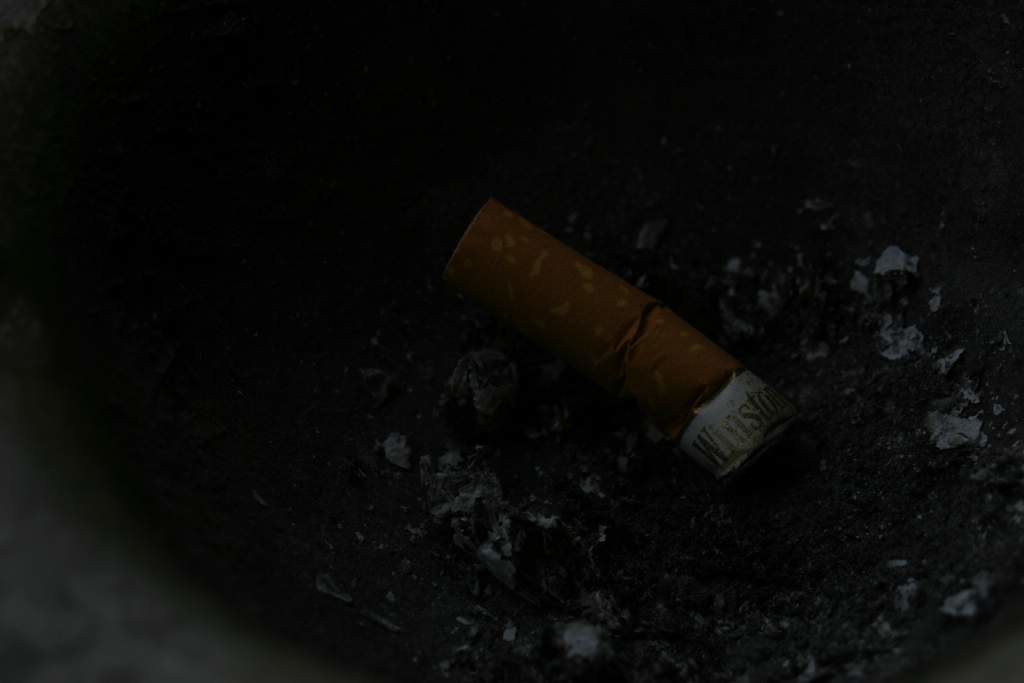In this close-up photograph, we see a discarded cigarette butt resting in a receptacle filled with grey and black ash, presumably from other cigarettes. The butt, with its orange filter, features various lighter orange spots and is slightly bent in the center. A white band wraps around it, bearing the brand name "Winston" in gold lettering. The cigarette is missing its main body, showing burnt marks on the white end, indicating it has been used. The receptacle's metal rim is visible in the bottom left corner, but shadows and darkness obscure further details about its structure, emphasizing the neglected lone cigarette butt amid the ash.